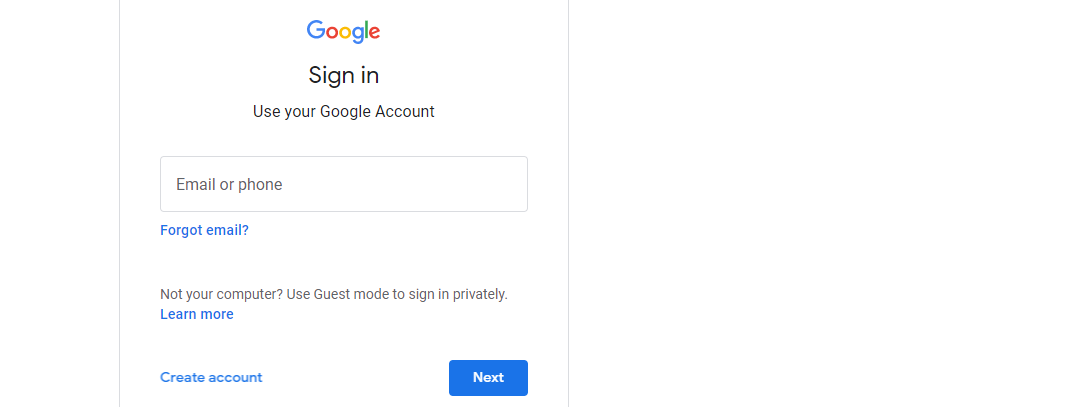The image depicts a Google sign-in page with a visually structured layout. The central feature is a white box framed by a gray border on its left, right, and top edges. Prominently positioned at the top center of this box is the colorful Google logo, comprising two blue G's, a red O, a yellow O, a green L, and a red E. 

Directly beneath the logo, the text "Sign in" is displayed, followed by the instruction, "Use your Google Account." Below this, there is a white rectangular textbox outlined in gray, with the placeholder text "Email or phone" situated towards the left inside the box. A blue hyperlink reading "Forgot email?" is positioned underneath the textbox.

Further down, after some spacing, a gray text states, "Not your computer? Use Guest mode to sign in privately," accompanied by another blue hyperlink that prompts users to "Learn more."

Following additional spacing is a blue hyperlink labeled "Create account." Adjacent to this, on the right side, is a blue rectangular button with the word "Next" written in white text at its center, indicating the option to proceed.